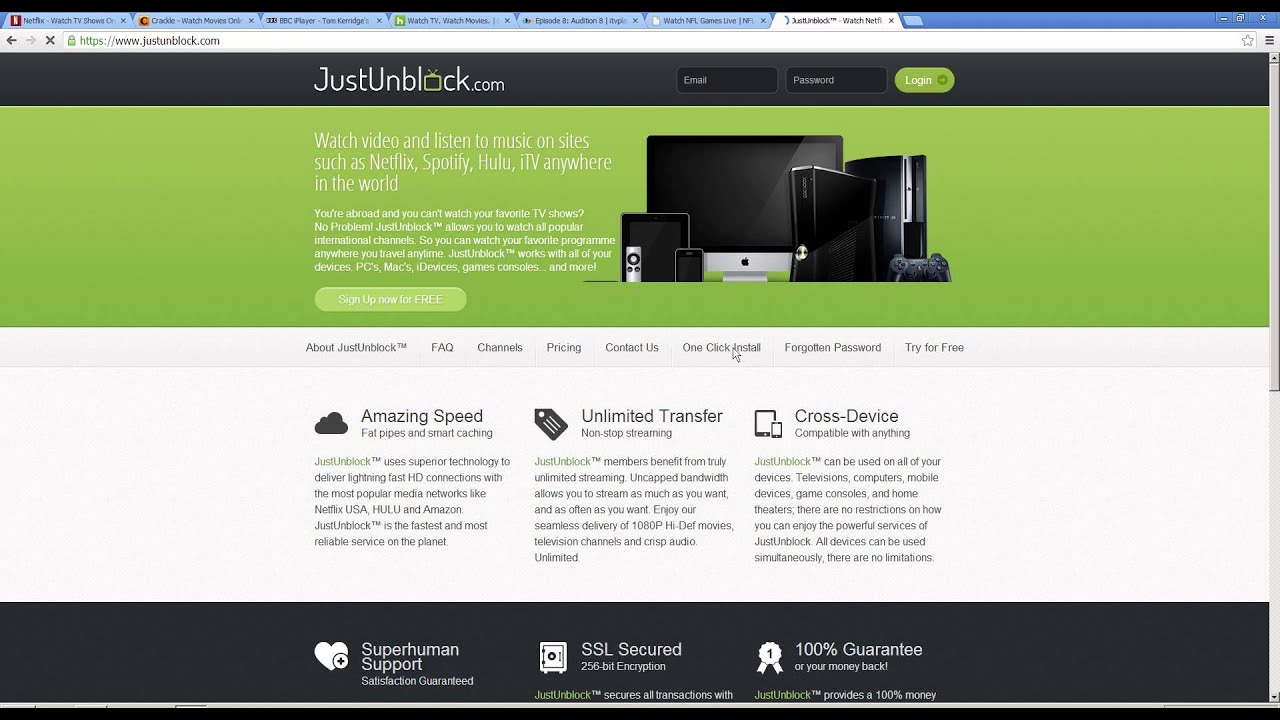### Descriptive Caption:

The image displays a detailed web page for "Just Unblock," a service promoting access to international channels and content streaming. At the top, multiple browser tabs are visible:

1. **Netflix**: The tab showcases a red box with a white "N" logo and a truncated text "Netflix: Watch TV shows on...".
2. **Crackle**: An orange square with a black "C" and partial text "Watch movies only...".
3. **BBC iPlayer**: A black rectangle with white "B", "B," "C" letters, and incomplete text referencing Tom Kerridge.
4. **Hulu**: Identified by a green square with a white "H" and text mentioning "Watch TV, Watch movies".
5. **ITV**: Featuring partial identification, with incomplete text "Episode 8 Audition" and "Watch NFL games live".

The primary web page being viewed is "Just Unblock." The interface has:

- **Header**: Dominated by a large black bezel. The site’s logo includes a green TV with rabbit ears.
- **Login Section**: Two black rectangles for email and password input, alongside a green login button with an arrow.
- **Device Icons**: Apple Macintosh, iPad, iPod, an Android tablet, Xbox 360, and a PS3, indicating supported devices.

The background is light green, complemented by multiple sections of white and black text:

- **Informative Text**: Describes service features such as watching video and listening to music on sites like Netflix, Spotify, Hulu, and ITV worldwide. Encourages users to try "Just Unblock" for unrestricted access to international TV shows.
- **Sign-Up Prompt**: A light green clickable button labeled "Sign Up Now for Free".

Additional buttons in a light gray bezel offer navigation options: About, FAQ, Channels, Pricing, Contact Us, One-Click Install, Forgot Password, and Try for Free.

Other elements include:

- **Support Features**: "Superhuman Support" alongside an icon of a heart and "SSL Secured 256-Bit Encryption."
- **Guarantee Ribbon**: Promising "100% Guarantee or Your Money Back".

Below, there is information about streaming speed and caching technologies, with claims of providing "lightning-fast HD connections" and "uncapped bandwidth." Visual icons represent cross-device compatibility with tablets, smartphones, PCs, game consoles, and home theaters, emphasizing unlimited and simultaneous use on multiple devices.

In summary, this web page for "Just Unblock" pitches a comprehensive streaming service for accessing global media content seamlessly across various devices.